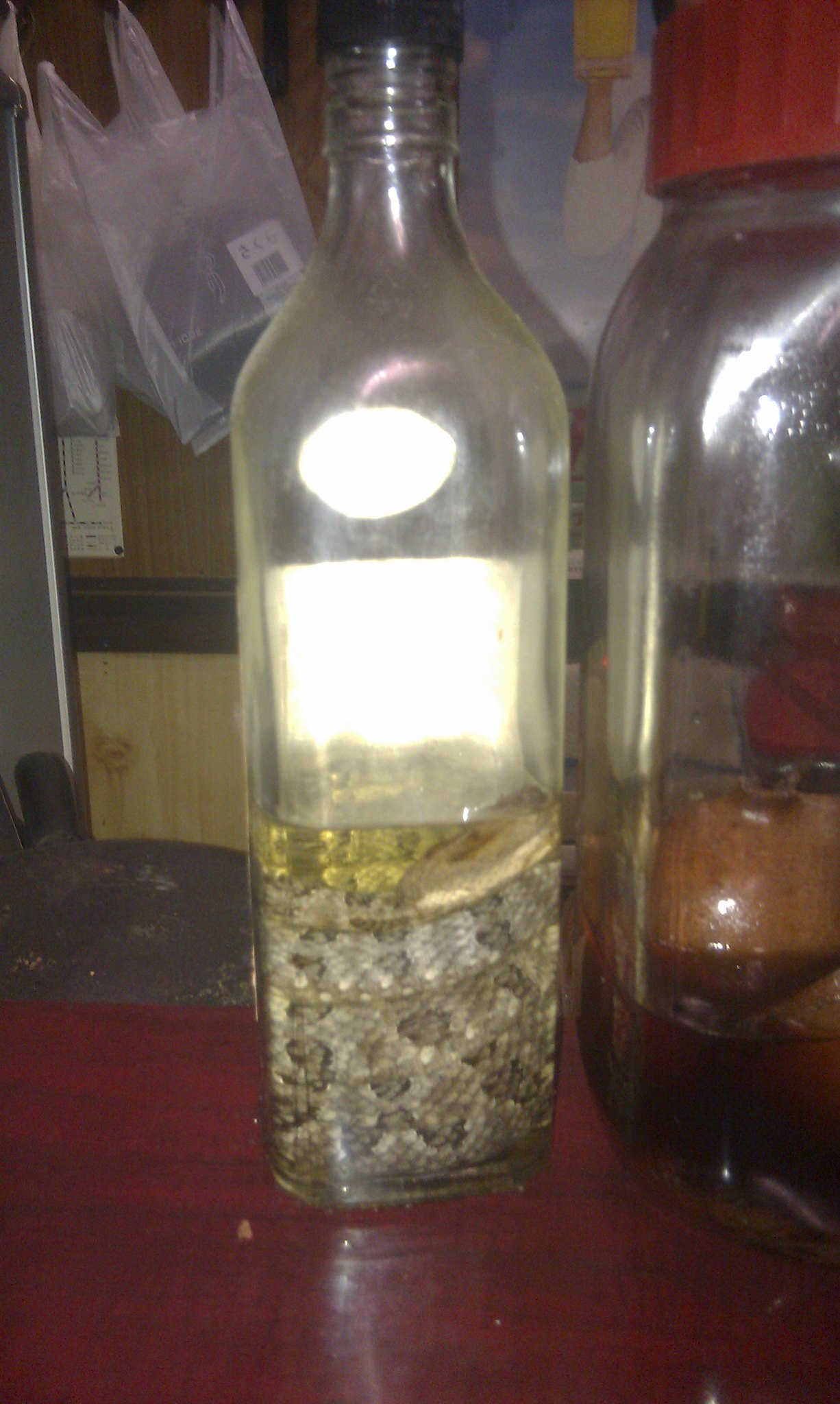This is an image depicting a scene with two distinct bottles placed on a reddish-brown wooden shelf or table. The primary bottle, reminiscent of those used for wine or vinegar, has a weathered appearance with a black cap and is partially filled with a mostly clear liquid. Inside the liquid, a brown and grey rattlesnake is coiled up at the bottom, evoking similarities to snake wine found in places like Vietnam or South America. Positioned beside this bottle is a typical oblong jar, capped with a red lid. The jar is similarly filled about a third of the way with a brown liquid, although the contents within are indiscernible. Behind these bottles, a bulletin board adorned with various pinned items, including plastic bags containing what appears to be dark clothing material, forms the background of the scene.